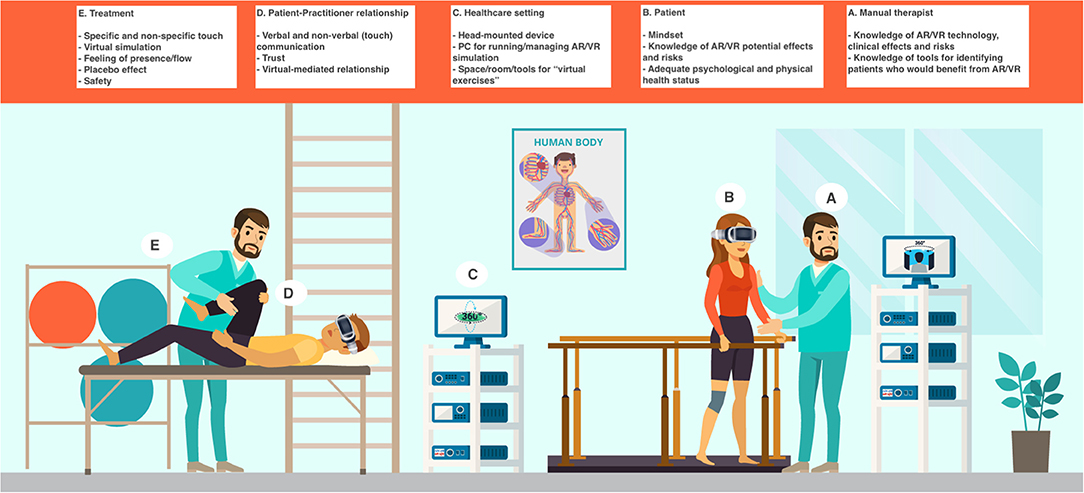The image is a diagram depicting patients in a physical therapy setting utilizing virtual reality technology. At the top of the diagram, white squares sequentially labeled A through E provide explanatory details. Below this, the image is rendered in an animated style. On the right side, a female patient is shown on an elevated platform with railings, akin to a treadmill, while wearing a VR headset. She is being assisted by a man in teal scrubs who also has a full beard and short hair. To the right of the female patient, a monitor is visible. On the left side, a male patient is lying on a table with his knee bent, also wearing a VR headset. He is being aided by another bearded, short-haired man in teal scrubs. Adjacent to the male patient, there is another monitor. This diagram appears to illustrate a futuristic medical facility, emphasizing the integration of virtual reality in therapeutic practices and detailing the interaction between patients and practitioners.